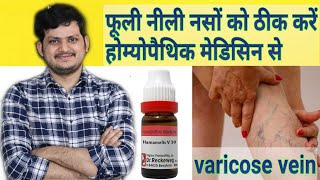This advertisement, likely in a Middle Eastern script, promotes a medication for varicose veins. The center of the ad features a brown, slightly see-through bottle with a white cap edged in red, although the text on the bottle is too small to read. To the left of the bottle stands a man wearing a black-and-white or dark-blue-and-white plaid shirt, his arms folded, and smiling confidently at the viewer. To the right, the words "varicose vein" are emblazoned in green above an image of a person gripping their leg, clearly displaying prominent varicose veins. The person's hand, adorned with red nail polish and showing visible wrinkles, further emphasizes the condition being treated. The layout and multilingual text suggest the ad is intended for a diverse audience, promoting the efficacy of the medication.